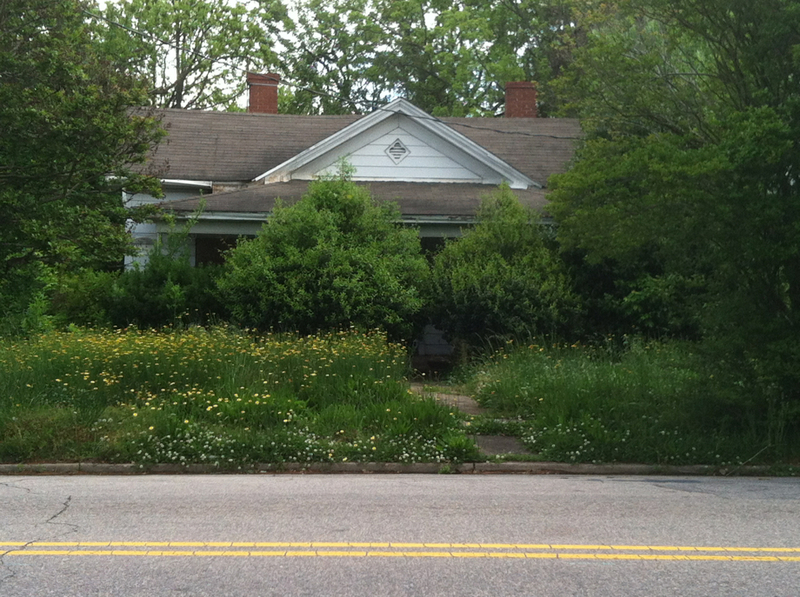In this image, an abandoned house is depicted across the street directly in our view. At the very bottom of the image, a light gray road with two yellow lines in the center, indicating separate lanes, runs horizontally. Just beyond the road is a gray curb, leading to a stretch of long, green grass dotted with sporadic white and yellow flowers on the left-hand side.

A section of a light gray walkway can be seen on the left side of the image, leading towards the house. The house is partially obscured by two trees standing in front of its entryway, as well as additional trees that line both sides and the background of the house. These trees are a dense, dark green color, adding to the overgrown and abandoned appearance of the scene.

The house itself features a gray roof and a white upper-level facade. Two red brick chimneys rise from the roof, further contributing to the aged and deserted aesthetic of the property. The overall composition conveys a sense of neglect and nature reclaiming the space.